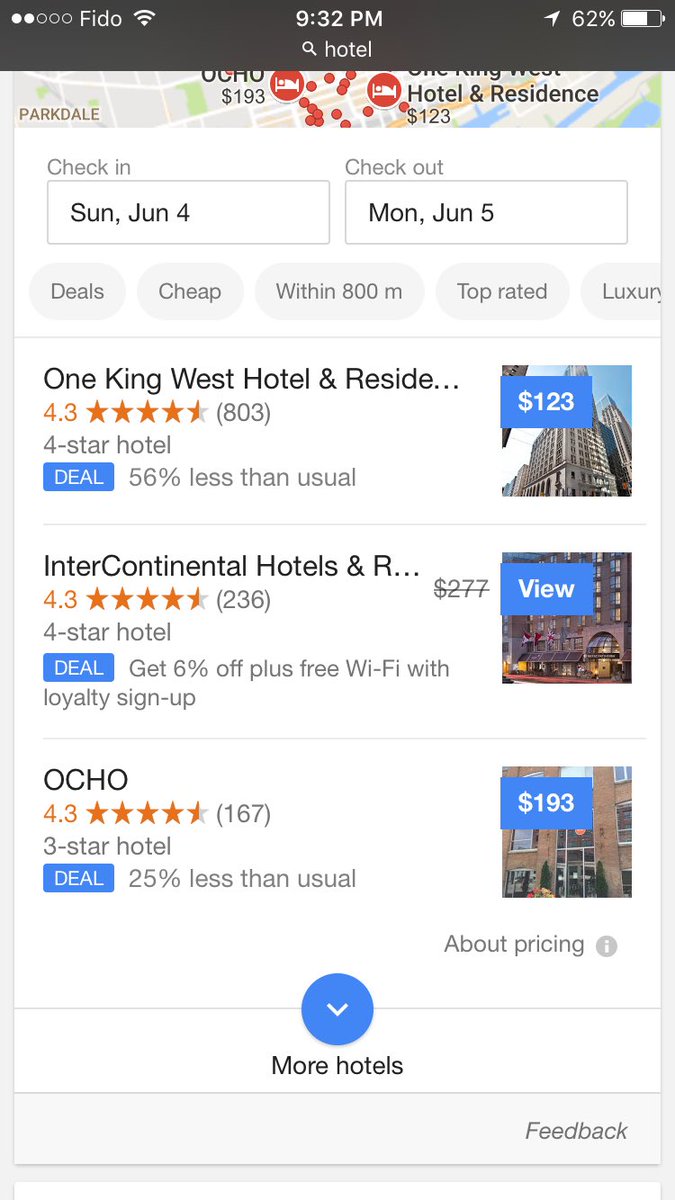The image displays a phone screen showcasing various hotels. At the top, a dark gray search bar prominently features the word "hotel." Just below the search bar, there is a partial view of a map marked with several red dots and two red circles, each indicating specific hotels along with their prices. Directly beneath the map, dual rectangular fields show check-in and check-out information: Check-in is set for Sunday, June 4th, and check-out for Monday, June 5th. Following this, a row of menu buttons in light gray with dark gray text offers options such as "deals," "cheap," "within 800 miles," "top rated," and "luxury."

The bottom section of the screen lists three hotels, each separated by thin gray lines. On the right side of each listing, a small square photo of the hotel is displayed, with the price highlighted in a small blue rectangle superimposed over the photo. To the left of each photo, the hotel's name is listed, accompanied by its star rating and available deals. This detailed arrangement provides a comprehensive overview of hotel options, making it easier for users to compare and select their accommodations.